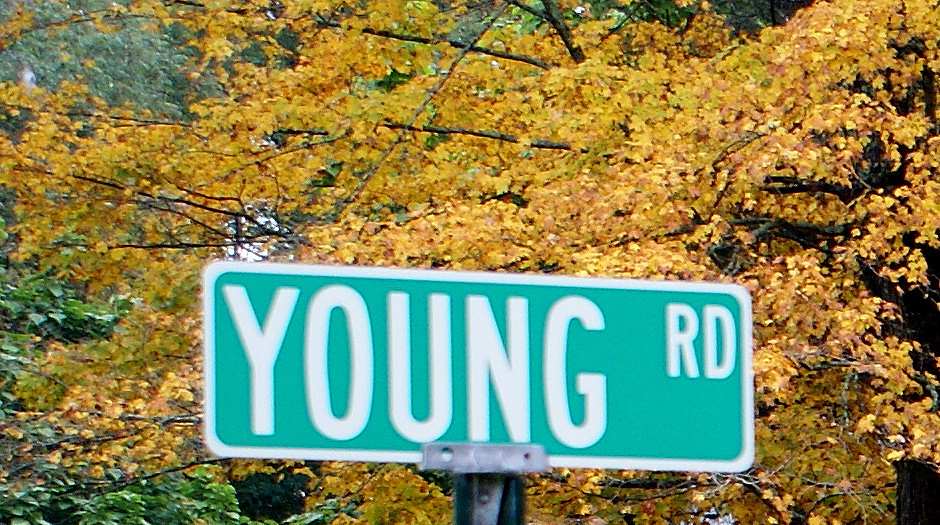The photograph features a rectangular, green street sign with a white border that reads "Young Road" in white letters, with "R-D" abbreviated in the top right corner. The sign is mounted on a silver metal post, with only the top portion of the post visible. The background is dominated by a striking mix of autumnal foliage and verdant greenery. In the foreground, a tree bursting with small, vibrant yellow leaves is prominently displayed, interspersed with a few bare branches. On the left side, greener trees are visible, their foliage still largely intact with no bare branches. To the right of the yellow-leaved tree, a large, dark black tree trunk provides a stark contrast. A hint of light blue sky peeks through the dense canopy, adding an extra layer of depth to the vibrant scene. Additionally, a green bush or tree is partially visible in the bottom left corner of the image.